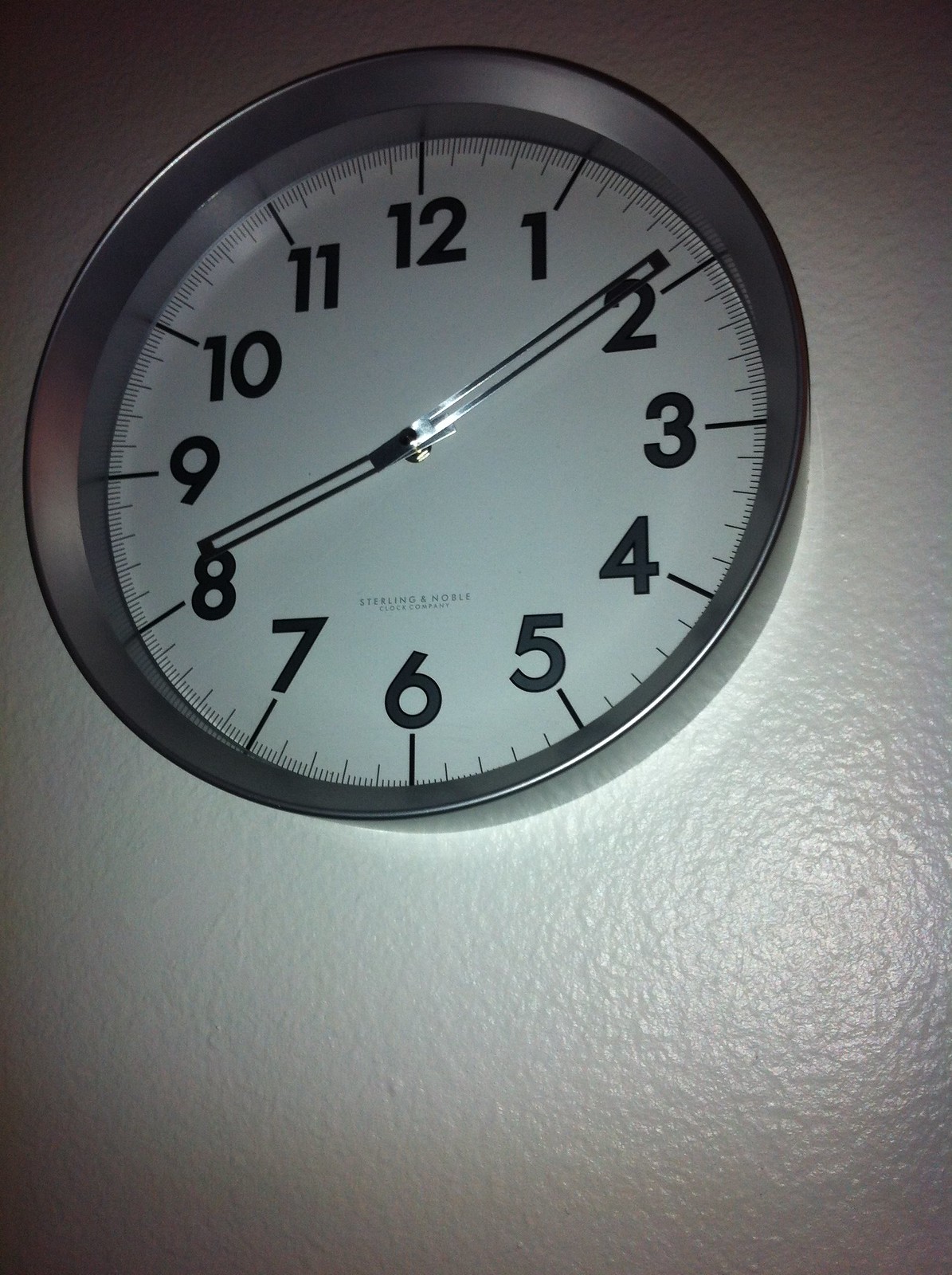The image captures a silver-framed wall clock mounted on a lightly textured white wall. The clock features a white face with bold black numbers from 1 to 12. The silver clock hands, unique in design with squared tips and a long hole in the center, indicate the time as 8:09. The photograph appears to have been taken in low light, with a flash illuminating the clock and creating contrasting shadows on the wall. The setting, likely indoors, presents the clock prominently, with the play of light and shadow giving the scene a slightly dramatic effect.